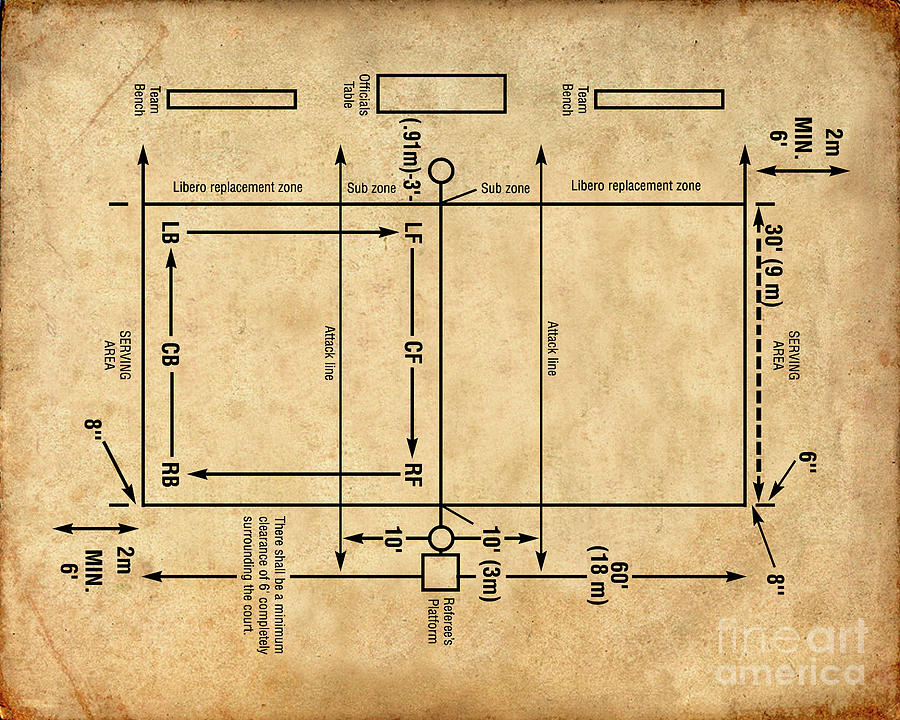Displayed on aged, light brown paper with dark brown, almost rust-colored edges, this detailed schematic resembles a volleyball court. Black lines and arrows are precisely printed across the worn, sideways paper, detailing various marked zones and their measurements. The top section features three labeled rectangles: "team bench" on both the left and right sides, and "officials table" in the center. The court's layout includes prominently labeled areas like "serving area," "libero replacement zone," and "attack line," repeated multiple times to emphasize their importance. Additional notations include measurements such as "30 feet," "9 meters," "6 inches," and "8 inches," ensuring exact dimensions of the court's elements. The bottom right of the schematic is marked with "fine art America," indicating its artistic representation, blending precise sports court design with an antiquated aesthetic. A minimum clearance of six feet completely surrounds the court, highlighting its functional and regulatory aspects.